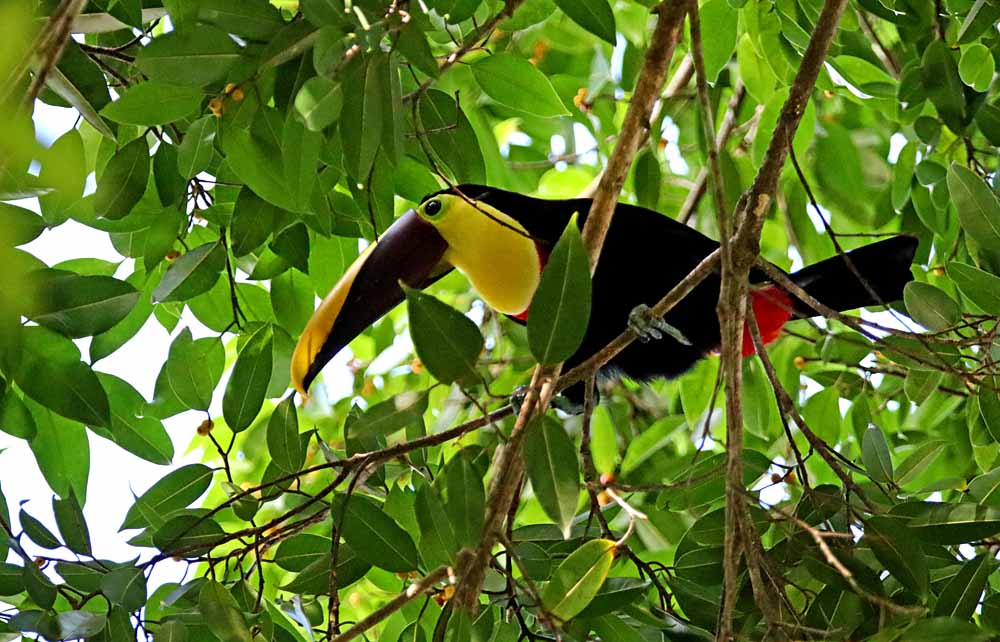In this vibrant photograph, a striking tropical bird is perched on a slender brown tree branch amidst lush green, oval-shaped leaves. The bird presents a captivating palette: predominantly black plumage with a vivid yellow face, a distinctive long beak that is yellow on top and dark brown on the bottom, and a splash of red connecting its body to its black tail. The side profile reveals the bird looking intently towards the left, with sunlight filtering through the dense foliage, casting soft, dappled light and revealing glimpses of the blue sky beyond the canopy.